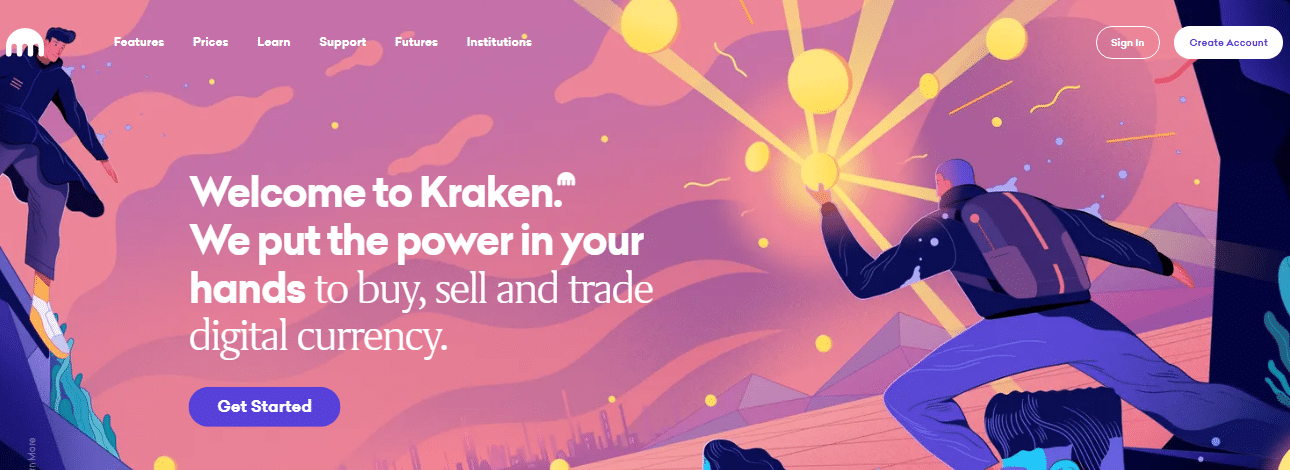The image features a stylish and visually engaging layout with a white top section displaying navigation links in white text: "Features," "Prices," "Learn," "Support," "Futures," and "Institutions." Below this is a large, vibrant rectangle that transitions from shades of purple to pink. 

On the left side, there is a whimsical, cartoonish illustration of a mountain scene. A person is depicted climbing the mountain, wearing a long black coat, purple pants, and white tennis shoes; a small white emblem is visible on their shoulder. The mountain itself is a blend of purple and turquoise hues, with a sky in the background painted in shades of pink and purple. 

In the foreground, another cartoon figure is shown from the back, wearing purple pants, a black long-sleeve jacket, and a purple backpack. This figure is holding up a large, sunburst-shaped object, depicted as a big yellow circle with radiant yellow stripes emanating from it. In the background, faint cityscapes and more mountains are visible, adding depth and context to the scene. Various streaks of graffiti-like elements adorn the sky, injecting a sense of urban artistry.

In the upper-right corner, a white-outlined banner prominently says "Sign In," and below it, a white banner with purple text reads "Create Account." Centered within the image, bold white text welcomes viewers with the message: "Welcome to Kraken. We put the power in your hands to buy, sell, and trade digital currency." Further down, a purple banner with white text encourages action with the phrase "Get Started."